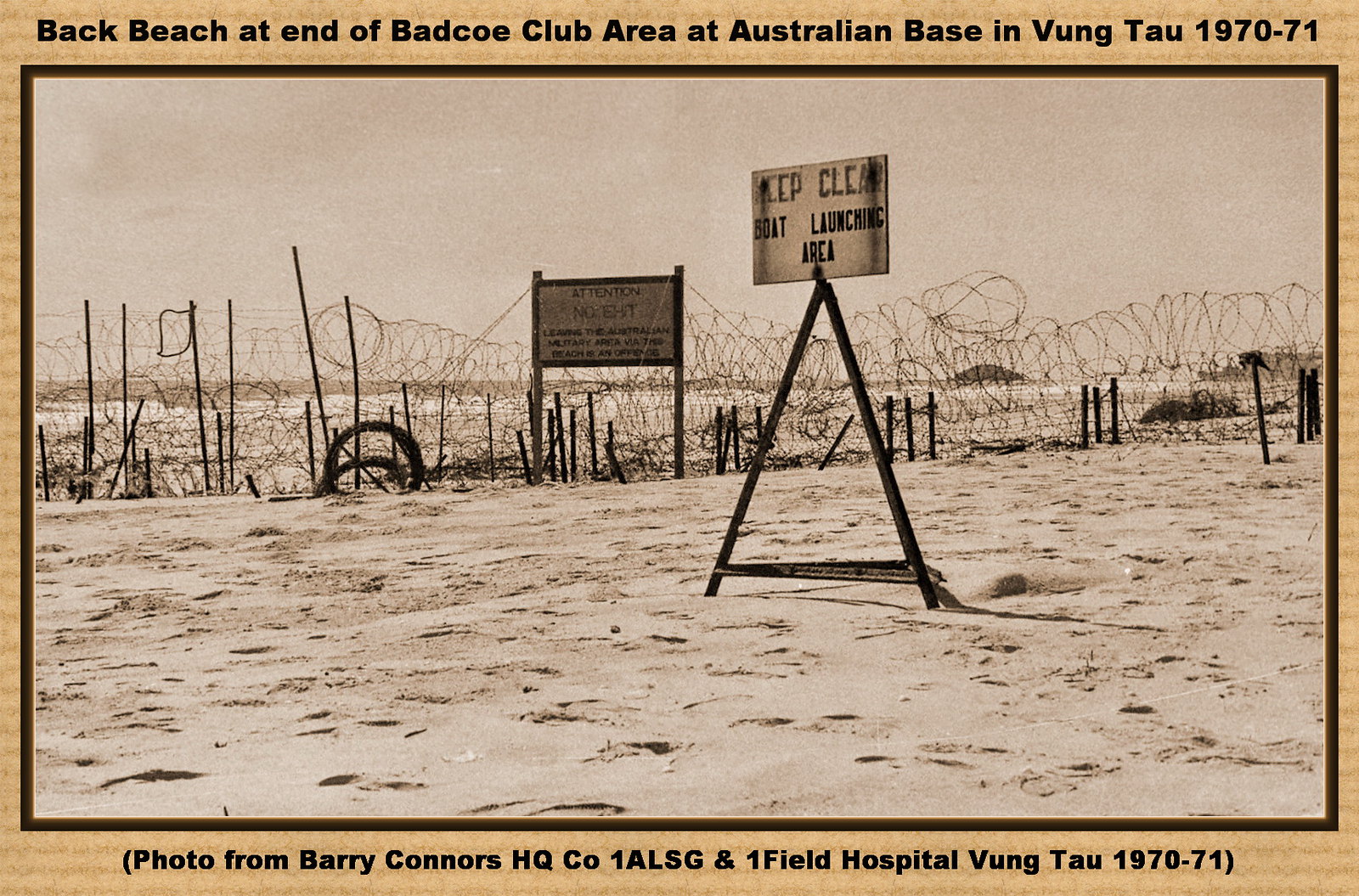This black-and-white photograph, meticulously bordered in beige, features a comprehensive header: "Back Beach at End of Bad Co. Club Area at Australian Base in Vung Tau, 1970 to 71." The image captures a sandy terrain, intersected by a barbed wire fence and additional coiled barbed wire in the background. Prominently featured are two signs; while one remains unreadable, the other, mounted on a tripod, clearly instructs, "Keep Clean Boat Launching Area." Below the image, a subtitle adds context: "Photo from Barry Connors HQ Company, One ALSG and Field Hospital, Vung Tau, 1970 to 71." This evocative snapshot offers a glimpse into a specific locale within the Australian military base during the Vietnam War era.